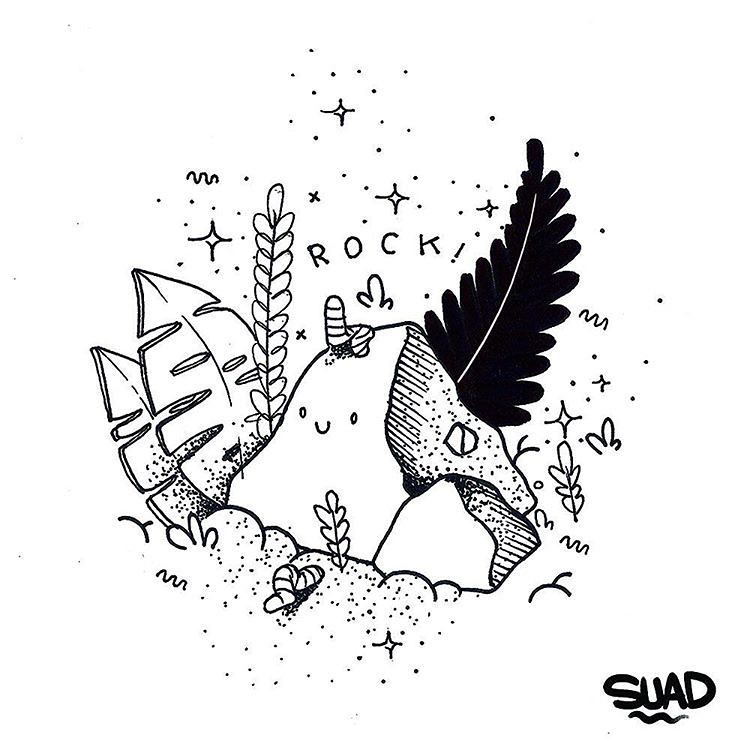This detailed black-and-white cartoon sketch features a central rock with a whimsical face, complete with two small, rounded eyes and an upwardly curving half-circle smile. The rock's left side appears flat, and on its right side, thin vertical lines extend downward with many tiny black specks scattered across its surface. At the very top of the rock, a small, squiggly worm emerges, while another worm burrows into the soil beneath.

To the bottom right of the primary, larger rock is a smaller rock of a similar shape. In the background, directly behind the larger rock on the right, a black bush, resembling a feathery or Christmas tree-like shape with a distinct white line in its center, extends upward. 

On the left side of the larger rock, a stick with leaves grows upwards. These leaves have intricate slits along their sides and are speckled with tiny black spots at their base. Two additional large leaves on the left side of the image appear more tropical, akin to palm tree leaves. Above the central worm, the handwritten word "rock!" is prominently displayed, surrounded by numerous small dots, stars, and whimsical drawings that pepper the sky above.

The artist, identified by the signature "S-U-A-D" at the bottom right corner, added a small squiggle beneath their name, completing this charming and nature-inspired doodle.